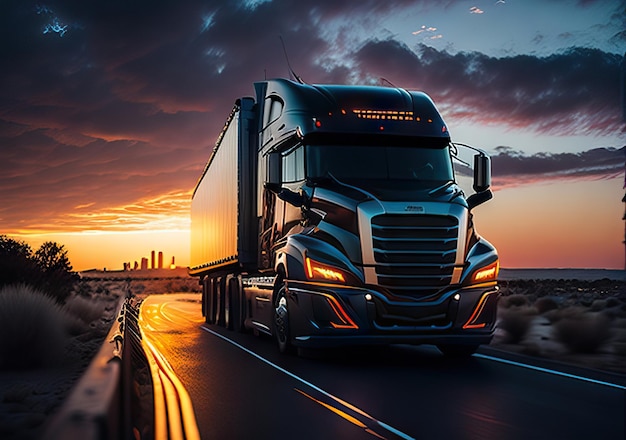This highly stylized image, potentially AI-generated or digitally enhanced, depicts a large, dark blue truck—possibly a 16-wheeler—driving along a solitary, hot highway at dusk or dawn. The truck, with its shiny, highly detailed grill and headlights that glow a soft orange, is centrally positioned, facing slightly to the right. The sun, either setting or rising, casts an orangey-pink hue across the sky, creating a stunning backdrop of purples, blues, and soft pink clouds. The road, reflecting the sun's warm tones, is bordered by bushes and railings, emphasizing the single lane that accentuates the stylized nature of the scene. To the left of the truck, there's a somewhat unrealistic city skyline with about six buildings silhouetted against the horizon. Darker clouds roll above, adding depth to the evening (or dawn) sky, while a suggestion of birds punctuates the scene.